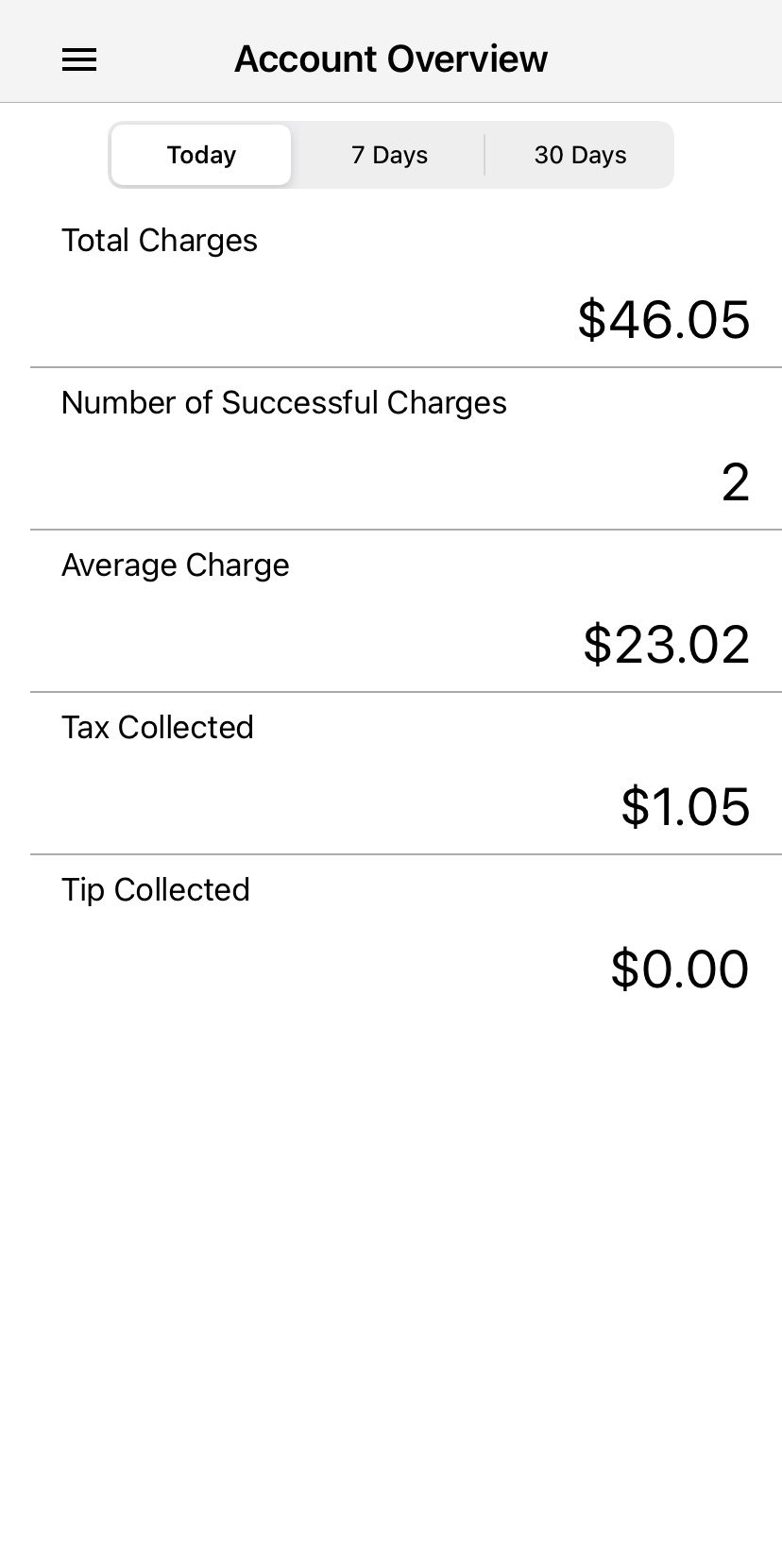This image displays a mobile or tablet screenshot of an accounting or financial tracking application. The interface features a white background. At the top, there is a gray bar with a black hamburger icon on the left, which typically indicates a menu for additional options. Adjacent to the icon, black text states "Account Overview."

Below this heading, three time-span options are lined up horizontally. The "Today" option is highlighted within a white rectangle, indicating it is currently selected, while the "7 days" and "30 days" options are in black text on gray rectangles.

Directly beneath these options, the screen provides various financial summaries. The first line reads "Total Charges: $46.05," followed by "Number of Successful Charges: 2." Next, "Average Charge: $23.02" is listed, with "Tax Collected: $1.05" and "Tip Collected: $0.00" following. Each financial metric has a dividing gray line to separate it from the next.

The layout and the detailed metrics suggest that this application could be used for financial accounting or business transaction tracking.